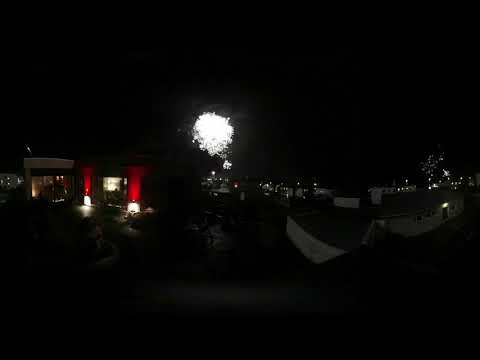The image captures a nighttime scene, shrouded in darkness, with a significant burst of bright white light in the center, resembling fireworks or a lightning bolt. This striking light punctuates the otherwise black sky, creating a focal point. In the foreground, slightly illuminated buildings and structures can be discerned. To the left, two pillars with white bases and red upper sections rise into the darkness, possibly framing an entrance. Beneath the illuminated sky, there are hints of street lighting from what appears to be storefronts, with white and red lights casting a glow. To the far right and under the light of the fireworks, more white buildings come into view, highlighting the architecture that is otherwise obscured by the night. The overall composition captures the contrast between the intense brightness of the fireworks and the deep black sky, with intermittent lighting revealing parts of the underlying cityscape.